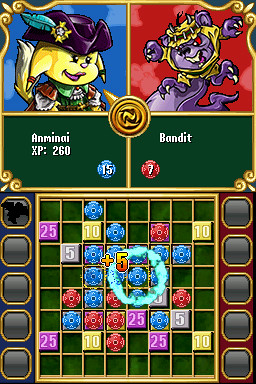This detailed caption was cleaned and formulated from the given text to provide a clear and descriptive overview of the image content:

---

This image is a screenshot from a mobile game, featuring a dynamic and visually engaging interface. At the top, two distinct characters are each enclosed in square frames with intricate golden ornate borders.

On the left side, there is a unique yellow, feminine creature with an unclassifiable appearance. It has a fox tail and is adorned with a dark purple western-style hat, which is embellished with a gold brooch and an elegant blue feather. The background behind this character is a gradient of blue shades.

To the right, a more intimidating purple monstrosity is depicted, characterized by its red eyes and menacing posture. This creature has four extended claws and wears a yellow hood with its ears protruding from it, set against a vivid red background.

Below these characters, two green sections detail their respective attributes. The left section, labeled “Anminai XP-260,” features a blue symbol, while the right section, labeled “Bandit,” showcases a red symbol.

Immediately beneath these descriptions is a grid layout bordered in gold, with green squares interspersed with numbered squares in purple, gray, and yellow. The grid also contains red and blue checkers, indicating potential player actions. An orange and yellow “+5” marker is prominent within this area, likely representing a recent game score update.

On either side of the main grid are four squares with gray interiors, framed with golden borders matching the background colors of the characters at the top. The top left square contains a silhouette of a bird, adding an additional layer of intrigue to the interface.

---